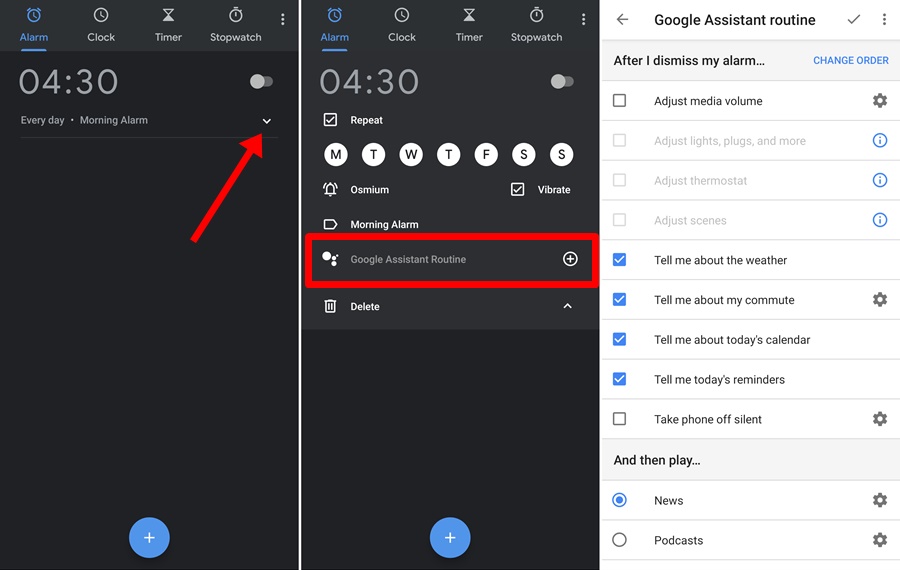A detailed and refined caption for the image described could be:

"This triptych showcases three screenshots of mobile applications. The two images on the left belong to the same application, featuring a consistent medium gray header. The header starts with a light blue alarm clock icon followed by light blue text reading 'Alarm,' which is underlined in the same light blue hue. Adjacent to this are white icons with corresponding white text: a clock labeled 'Clock,' an hourglass labeled 'Timer,' and a stopwatch labeled 'Stopwatch.' At the far right, three white dots are stacked vertically, indicating more options.

In the leftmost screenshot, the background beneath the header is black. The top left corner displays light gray numerals '04:30' with small light gray text underneath that reads 'Every Day,' followed by a dot and 'Morning Alarm.' In the top right, there is a light gray selection button in the shape of a pill, with an even lighter gray circle positioned on its left side. Below this, a white downward-pointing arrow is visible, overlaid with a bright red arrow emphasizing the white arrow. At the bottom center of this page, a blue circle with a white plus sign is evident.

The middle screenshot shows an expanded view of the alarm. Here, the same time and selection button are present, but under the time, there is a white checkbox with a checkmark. To its right, small white text reads 'Repeat.' Below this, white icons remain. Consistent with the first, the bottom also features the blue circle with the white plus sign.

The third screenshot, unlike the first two, has a white background with lines of black text, each line accompanied by a checkbox. This layout appears to include a list format, distinct from the alarm-focused interface of the previous two images."